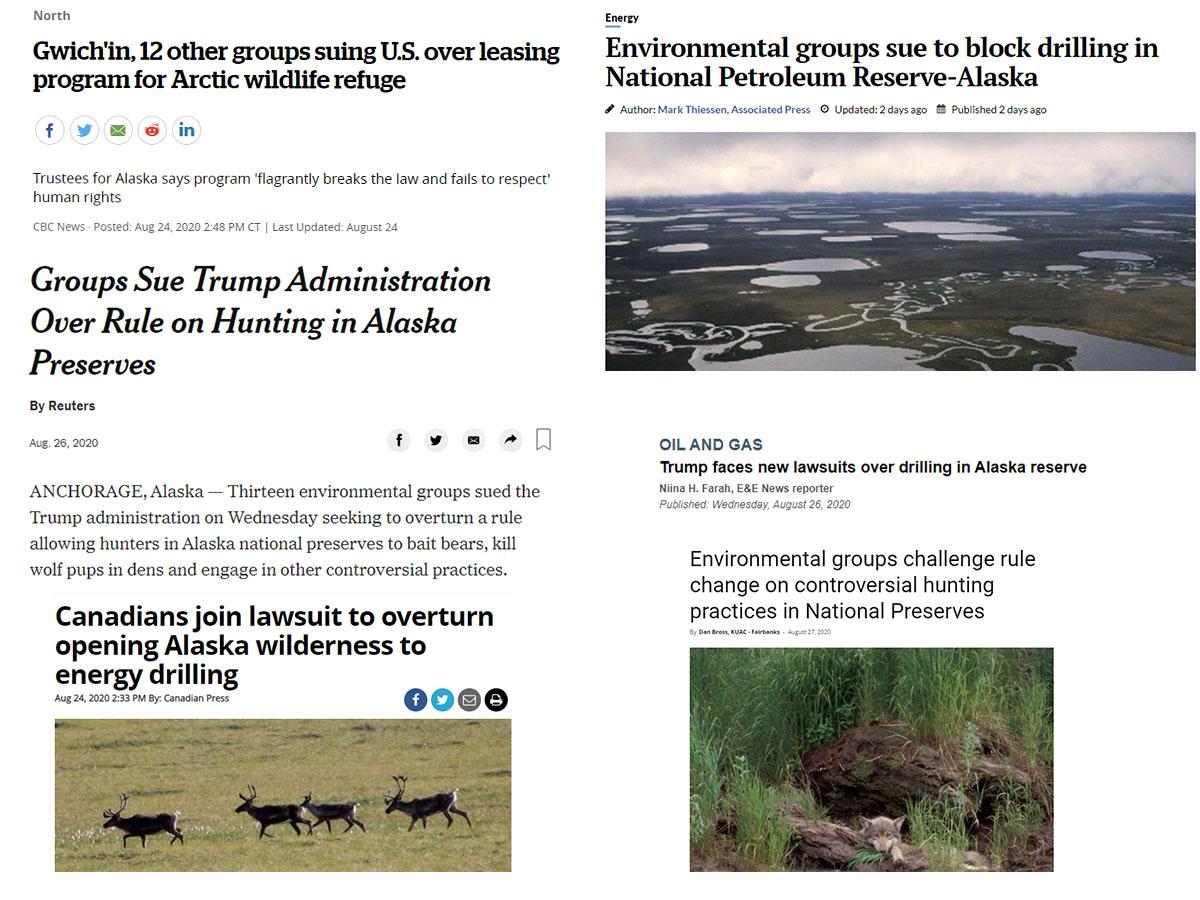**Caption:**

The image is a collage of news headlines, text snippets, and pictures, indicative of various reports concerning legal actions against the U.S. government over environmental and wildlife issues in Alaska. 

- **Left Column:**
  - **Headline:** "North Gwinnett's 12 other groups suing US over leasing program for Arctic wildlife refuge". 
    - **Below the headline:** Logos of social media and job platforms including Facebook, Twitter, email, Reddit, and Indeed.
  - **Subheadline:** "Trustees for Alaskan says program frequently breaks laws and fails to respect human rights".
  - **Another Headline:** "Groups sued Trump administration over rule on hunting in Alaska preserves" (by Reuters).
    - **Article Text:** "Anchorage, Alaska - 13 environmental groups sued the Trump administration on Wednesday, seeking to overturn a rule allowing hunters in Alaska preserves to bait bears, kill wolf pups in dens, and engage in other controversial practices."
  - **Further Headline:** "Canadians join lawsuit to overturn opening Alaska wilderness to energy drilling".
    - **Associated Image:** A picture depicting deer, caribou, or possibly elk.

- **Right Column:**
  - **Headline:** "Environmental groups sued to block drilling in National Petroleum Reserve's Alaska".
    - **Associated Image:** Pictures of lakes, presumably situated in Alaska.
  - **Further Headline:** "Trump faces new lawsuit over drilling in Alaska reserves".
    - **Subheadline:** "Environmental groups challenge rule change on controversial hunting practices in National Preserve".

The detailed compilation showcases the multifaceted legal actions taken by environmental groups and their international allies against the Trump administration's policies on wildlife management and energy drilling in Alaskan reserves, underscoring concerns about law violations and human rights.